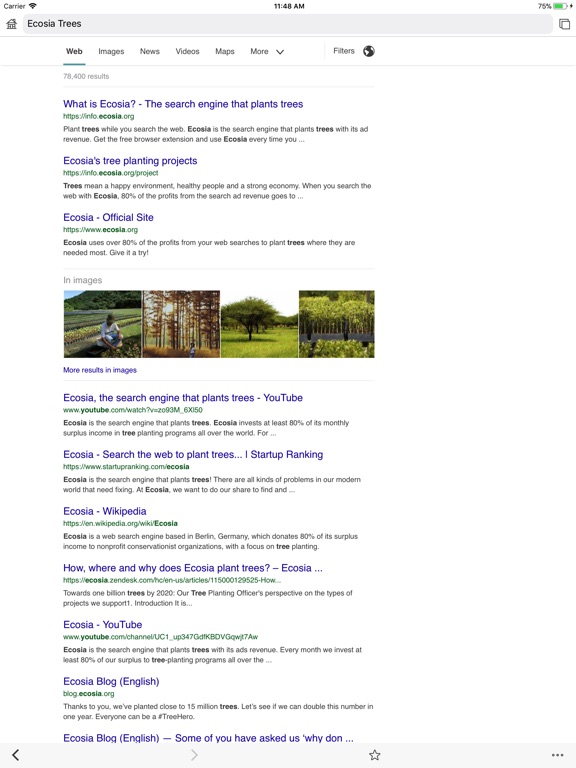This is a detailed screenshot capturing Google search results on a smartphone. At the top, the search query "Ecosia Trees" is prominently displayed in the search bar. Directly beneath, the Google search menu offers various filtering options, including Web, Images, News, Videos, Maps, and More, allowing users to refine their search type.

Following this menu bar, the search results for "Ecosia Trees" are displayed. The first three results are web links: "What is Ecosia?", "Ecosia Tree Planting Projects," and the "Ecosia Official Site." Below these links, there is an "In Images" section that showcases a preview of images for the search term "Ecosia Trees." The preview includes: a man planting a tree, a serene forest setting, a single tree in an open field, and lastly, an image depicting multiple planted trees in front of a fence, although the details of this last image are slightly unclear.

Continuing down the page, there are an additional seven web search results related to "Ecosia," providing further information and resources on the topic.